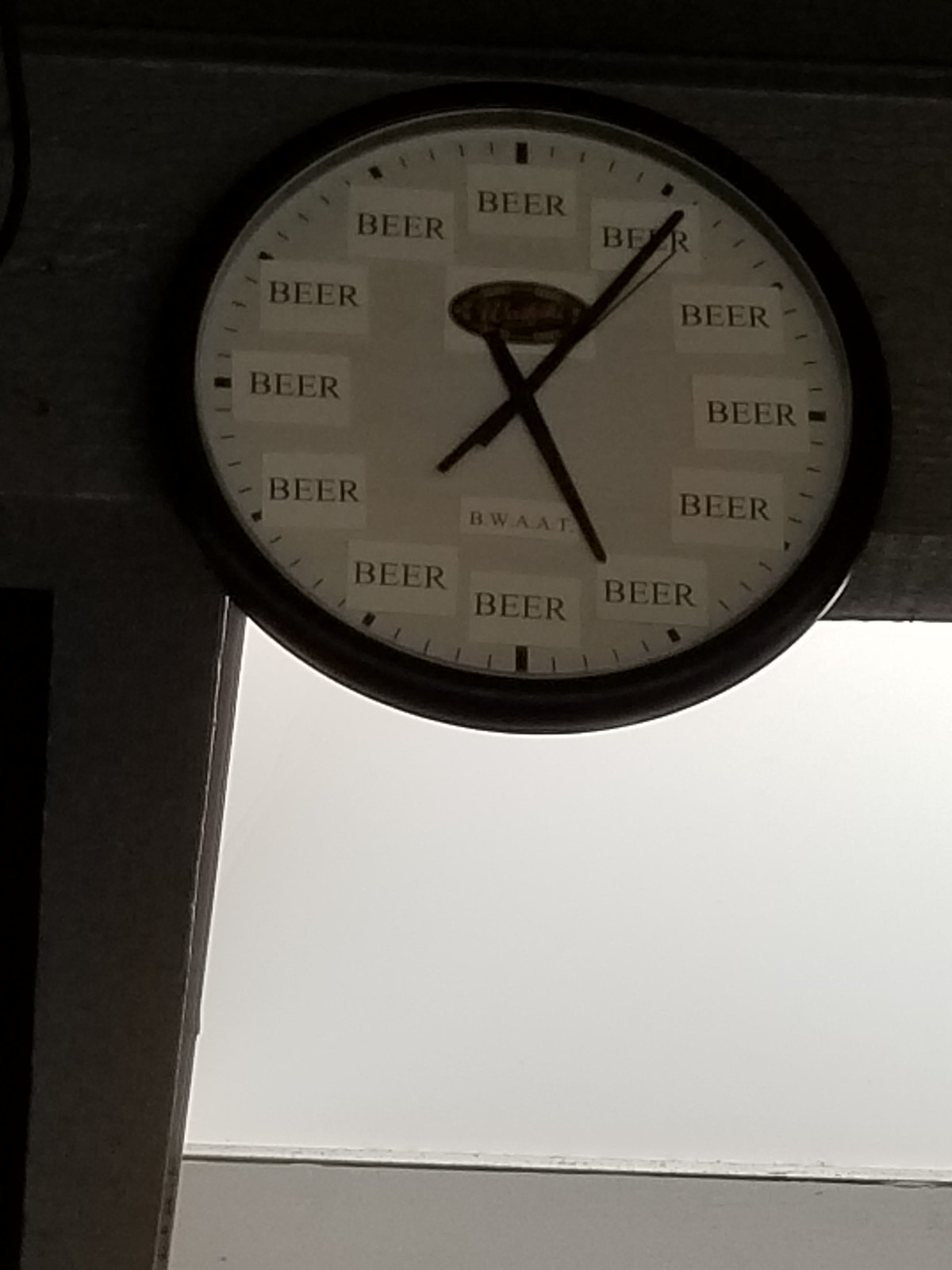A carefully framed color photograph captures a unique ornamental clock adorning a wall. The image predominantly features a black, white, and shades-of-grey palette, with a hint of beige lending a subtle warmth to the scene. This round clock, positioned prominently, boasts black hands set to five past five and a distinctive black logo at its center. Instead of conventional numerals, the clock face is adorned with white stickers, each bearing the word "beer" in black lettering, reinforcing the playful message that any time is perfect for a drink. The clock is mounted on what appears to be an exterior wall, with two distinct grey squares — one light, one dark — suggesting a transition from inside to outside. The surrounding environment is characterized by dark-toned walls and ceiling, emphasizing the clock's quirky and humorous design. Beneath the clock hands, a slightly obscured logo, possibly reading "smart" or "SWAT," adds an enigmatic touch to the overall composition.